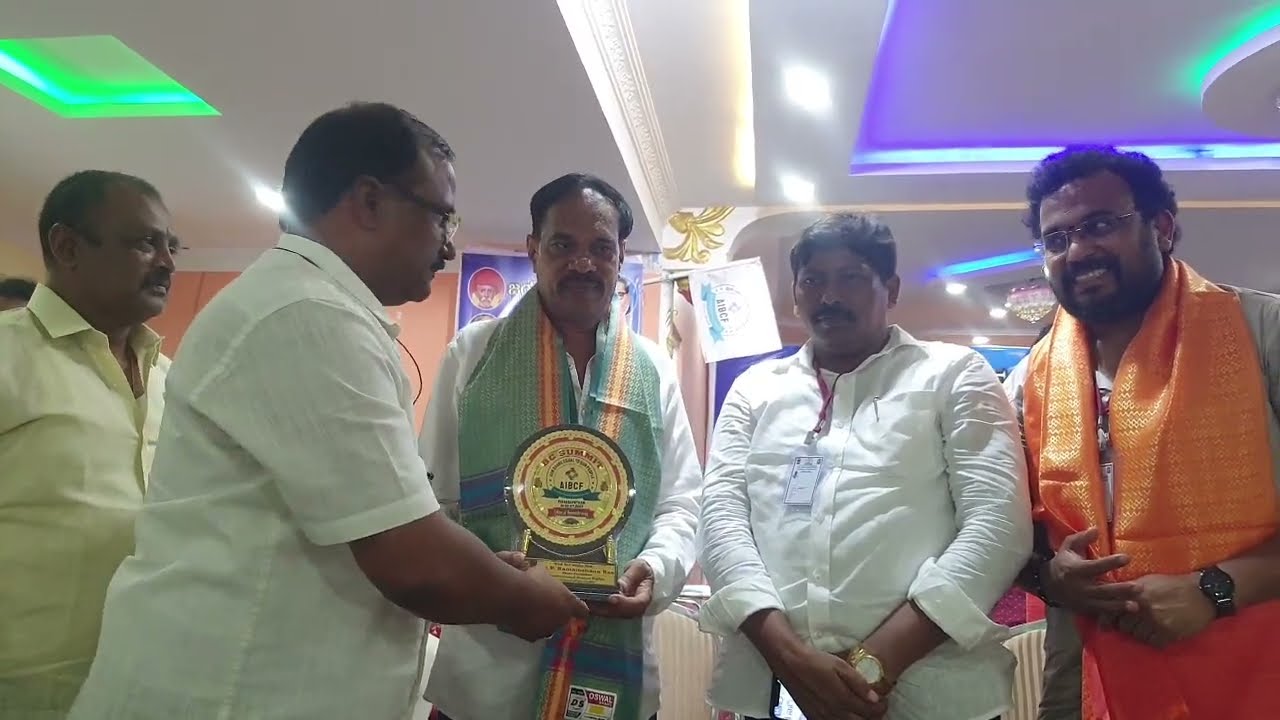In the center of the image, five gentlemen of Indian or Pakistani descent are gathered in what appears to be an indoor banquet or ballroom setting with overhead multicolored lights, including green and purple. One of the gentlemen, wearing glasses and a button-down shirt, is looking at another man who is receiving an award. The award recipient, also wearing a button-down shirt, has a green shawl with an orange and maroon stripe around his neck and is holding what seems to be a plaque. The other individuals, all sporting light-colored button-down shirts and dark skin tones, are either conversing or looking at the award presentation. Among them, a man on the far left wears glasses, and another on the far right, who has a short beard and mustache, is adorned with an orange shawl. Background elements include various wall hangings or flags and a chandelier, contributing to the suggestion that this event might be some sort of award ceremony or formal presentation. The backdrop is somewhat cluttered with posters and decor that are difficult to distinguish.